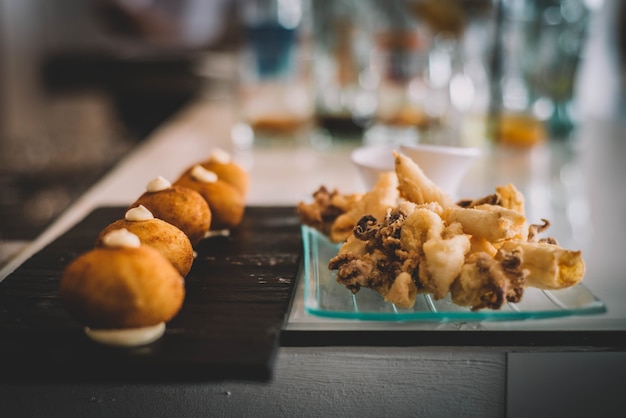The image depicts an array of pastries spread across a light brown countertop, resembling a bakery display. In the foreground, there are two distinct sets of pastries clearly visible. To the left, five cream puffs with dollops of white icing resemble small Hershey kisses on their dark brown surfaces, arranged neatly on a dark plate that slightly hangs off the edge of the table. On the right, a collection of thin, doughy, light brown pastries of various shapes and sizes are piled on a clear glass plate with cyan accents. Interspersed within this pile is a darker, frosted pastry with many curls. In the blurred background, the countertop extends further, featuring a line of mostly empty, clear coffee cups with remnants of various substances—brown, black, white, and orange—in them. Additionally, near the glass plate of pastries, there are two small white bowls resembling dipping sauce containers. The entire scene is set against a slightly grey backdrop, complementing the bakery-like ambiance.